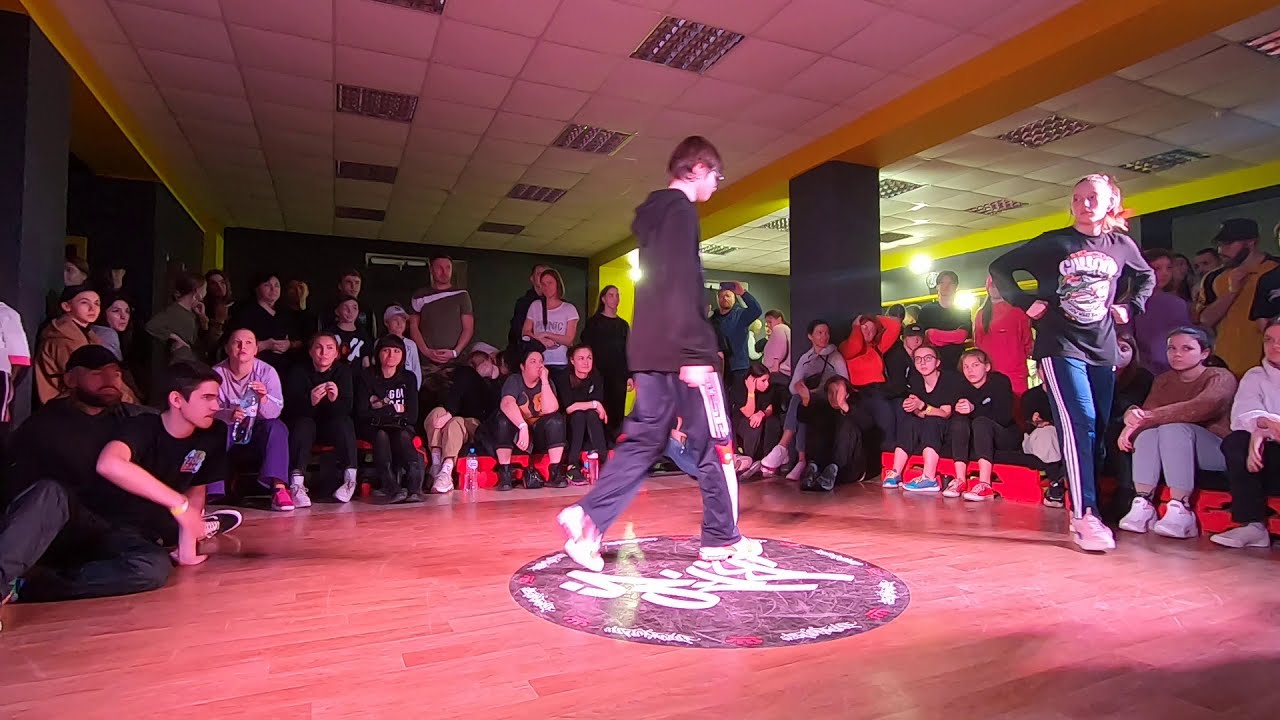The image depicts a young man, dressed in black sweatpants and a black sweatshirt, positioned at the center of what appears to be a dance studio with a wooden floor. He is clearly poised to perform a breakdance move, possibly a moonwalk, and he wears glasses. Surrounding him is a diverse crowd of spectators, mostly young people, some seated on the floor while others stand against the wall. A young woman, also in a loose, casual outfit similar to the man’s, stands nearby with her hands on her hips, suggesting she might also be a participant in the dance activity. The setting includes a circle with graffiti-like writing on the floor, hinting at a dance competition or demonstration, possibly involving a hip-hop dance troupe. The scene is lively, with the anticipation of an impending dance battle hanging in the air.